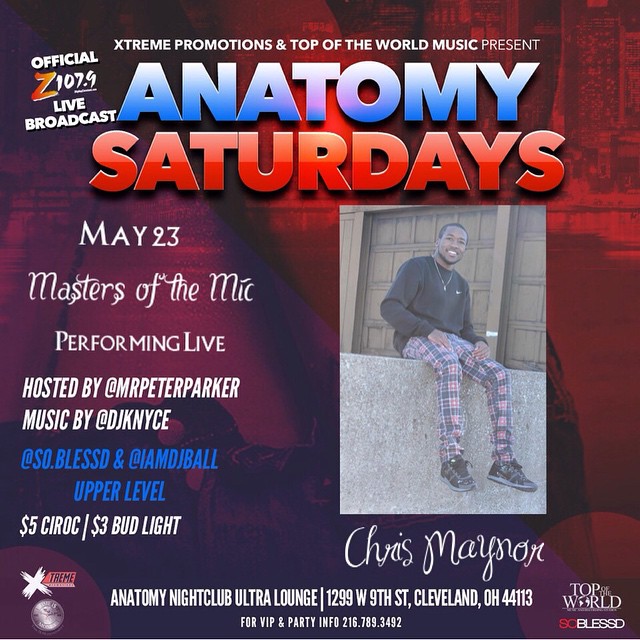This vibrant flyer promotes "Anatomy Saturdays," a live event happening on May 23rd at Anatomy Nightclub Ultra Lounge, located at 1299 West 9th Street, Cleveland, OH 44113. The event is brought to you by Extreme Promotions and Top of the World Music, featuring an official Z107.9 Live Broadcast. The headlining act "Masters of the Mic" will perform live, hosted by Mr. Peter Parker with music by DJ Nice. The flyer prominently features the title "Anatomy Saturdays" with "Anatomy" in blue and "Saturdays" in bold red font. A noteworthy detail is the $5 Ciroc and $3 Bud Light special mentioned. The lower part of the flyer showcases a man, Chris Maynard, dressed in a black long-sleeve shirt, plaid pants, and black shoes. The design is set against a red and purple background, and the bottom right corner displays "Top of the World," where "World" is depicted as a globe, followed by the phrase "So Blessed."